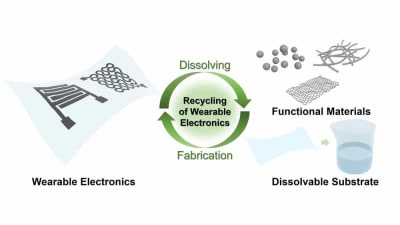This detailed illustration visually explains the recycling process of wearable electronics against a white background. Central to the image, two green arrows form a circle encapsulating the core concept. At the top of this circular arrow, the word "dissolving" is written in green, and at the bottom, "fabrication" is indicated. Enclosed within this circular arrow, against a green haze, the phrase "recycling of wearable electronics" is prominently displayed in bold black lettering.

To the left of the circle, there is a depiction resembling a flag that bears the words "wearable electronics." This flag features images of interconnected squares and a maze-like design of wires. To the right of the main circle, black text reads "functional materials," accompanied by a sequence of visual elements including dots, gray noodle-like shapes, and a mesh pattern.

Below these, another diagram shows a transparent beaker filled with a light blue liquid, and next to it, a piece of fabric with a green arrow pointing towards the beaker. This setup is labeled "dissolvable substrate" in black text.